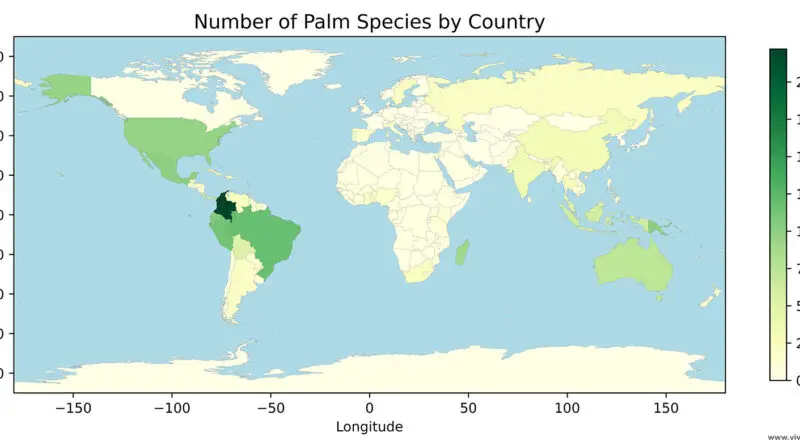This image is a detailed world map illustrating the number of palm species by country. At the top of the map, there's a title indicating "Number of Palm Species by Country." The map uses a color-coding system: dark green, green, light green, light tan, and white, to represent the density of palm species. Darker shades indicate a higher number of species, while lighter shades indicate fewer species or none.

The map spans all continents from negative 150 to positive 150 longitude, depicting detailed geographical distinctions. The United States, inclusive of Alaska, and Brazil are shown in green, indicating a relatively high number of palm species. Mexico also appears in light green, while Canada is not shaded at all, indicating no palm species. Similarly, mainland Africa is entirely white, reflecting an absence of these species.

In South America, Brazil and likely Colombia are shaded green. Russia is shaded in tan, whereas Australia is light green. Other notable color-coded regions include Greenland and Antarctica, both shown in yellow and tan respectively. Egypt and Japan are marked in white, while China is represented in tan. The oceans are displayed in blue, with most other countries either unlisted or color-coded accordingly.

Additional longitude markers are present at the bottom of the map, aiding geographical orientation. This comprehensive map provides an insightful visual representation of the global distribution of palm species.